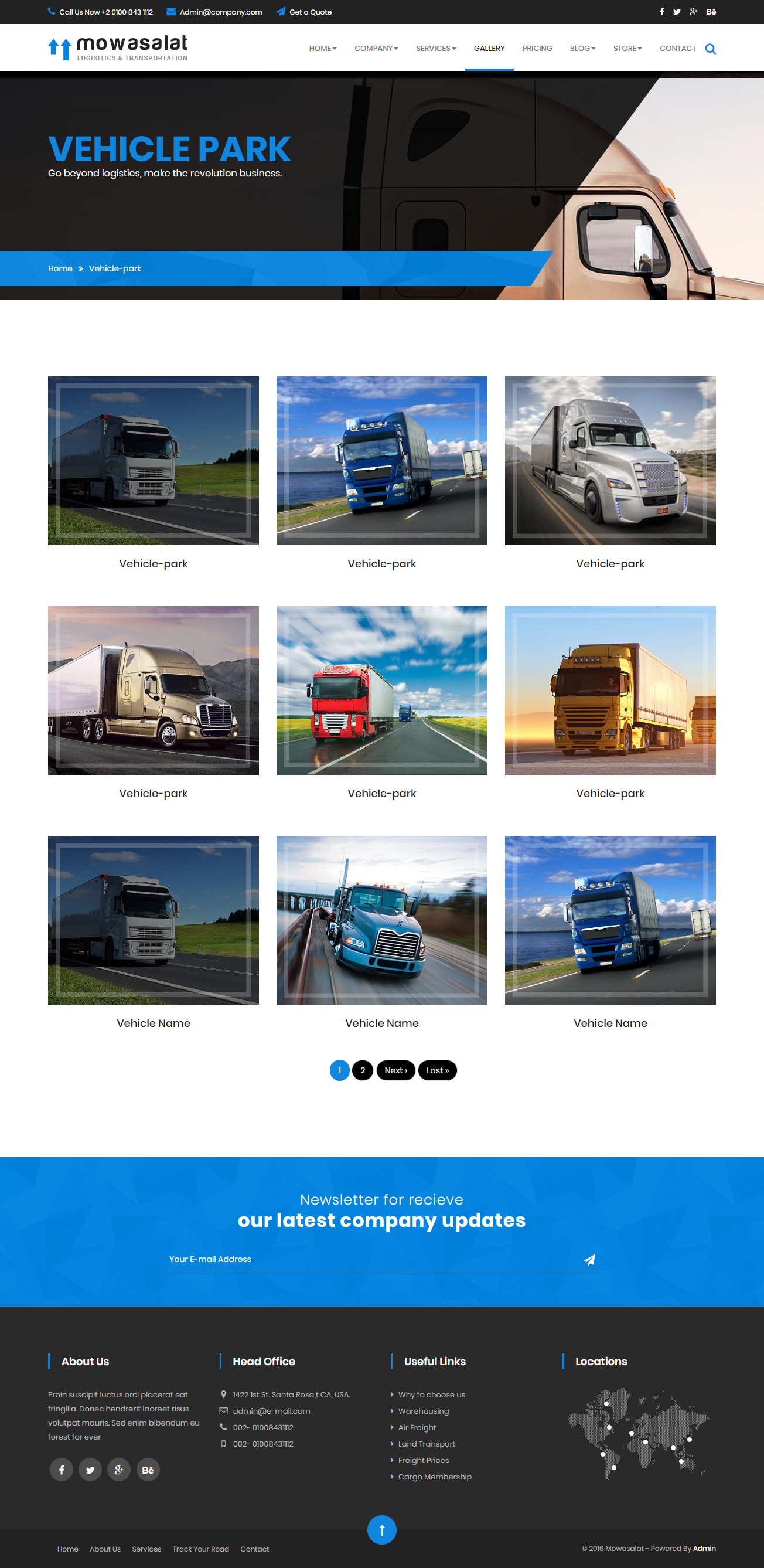**Detailed Caption:**

This image depicts a webpage from a company named "Moasalat," as indicated by its logo positioned at the top of the page. The header of the webpage includes standard browser control icons for maximizing, minimizing, and closing the window. Adjacent to the company name, there are several drop-down menu options, though the text is too small to decipher.

Beneath the header, the most prominent feature is a large blue banner with the words "Vehicle Park" superimposed on an image of a truck cab. Below the banner, the webpage displays a grid of nine images showcasing various types and sizes of trucks, including 18-wheelers. Each truck has a caption underneath, although the text is too small to read.

Further down the page, there are navigation radio buttons that allow users to scroll through the images. Below these buttons, the page seems to contain standard company details and updates, although the text remains unreadable.

At the very bottom of the page, a footer section includes several links, potentially for locations, company information, and social media profiles, but these details are also too small to make out.